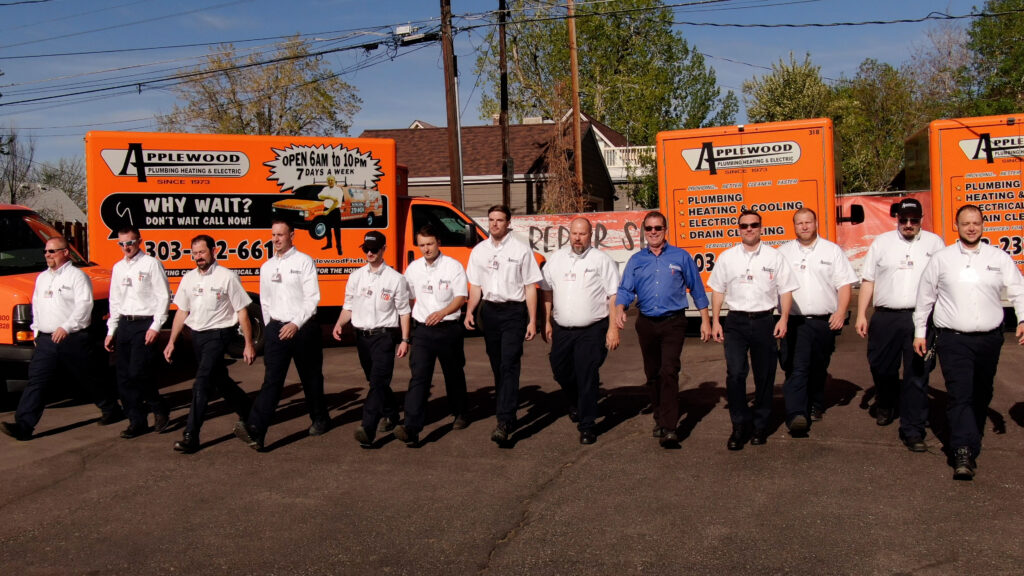The image depicts a team portrait of Applewood Plumbing, Heating, and Electric employees, taken outdoors on a clear, sunny day. A group of 13 men is walking towards the camera, spanning the width of the photograph. Out of these, 7 men on the left are dressed in white shirts and blue pants. The central figure, possibly a manager or a prominent figure in the company, stands out with his blue shirt, black pants, and sunglasses. To his right are 4 men also in white shirts but with black pants; two of them wear sunglasses, and one sports a hat. In the background, four distinct orange company trucks are visible, affirming the company’s identity. The first truck’s front end is visible on the left. Next to it, a truck parked sideways displays an advertisement for Applewood Plumbing Services, highlighting their operating hours from 6 a.m. to 10 p.m. and slogans "Why wait?" and "Don't wait, call now." Directly in front of this truck, another truck’s rear, bearing the company’s name and service details (plumbing, heating, cooling, electric, and drain cleaning), faces the camera. Finally, another truck's half rear is visible on the right, also marked with the company’s name and services offered. The team photograph is set against a backdrop that includes residential structures and trees.